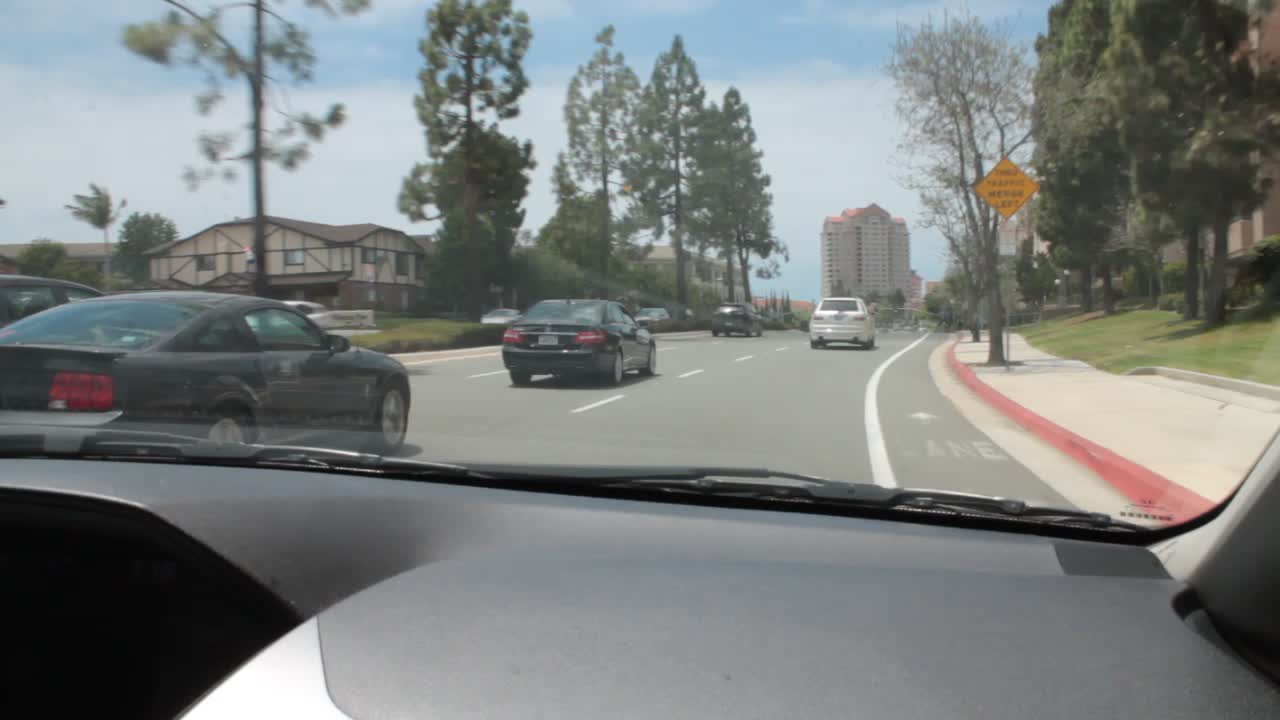Taken from the passenger seat of a car during daylight, this image captures the view through the windshield as the vehicle travels along a three-lane road. The car is positioned in the rightmost lane, adjacent to a narrow parking or bike lane. To the right of the vehicle, a sidewalk lined with light-gray concrete runs parallel, bordered by green, leafy trees, and a strip of grass.

In the opposite direction, a center median filled with grass and more trees separates the lanes of traffic. On the far left of the image, another set of lanes accommodates oncoming traffic, suggested by the presence of a white stucco house with a brown thatched roof in the distance and additional trees.

Directly ahead, a white minivan leads the vehicle, while to its left, another black car can be seen. A black hatch sedan drives adjacent to the car, with another black sedan visible in front of it. The car's interior, particularly the black windshield frame, does not reveal the make or model of the vehicle. The scene reflects a typical drive on a well-treed urban road during the day.